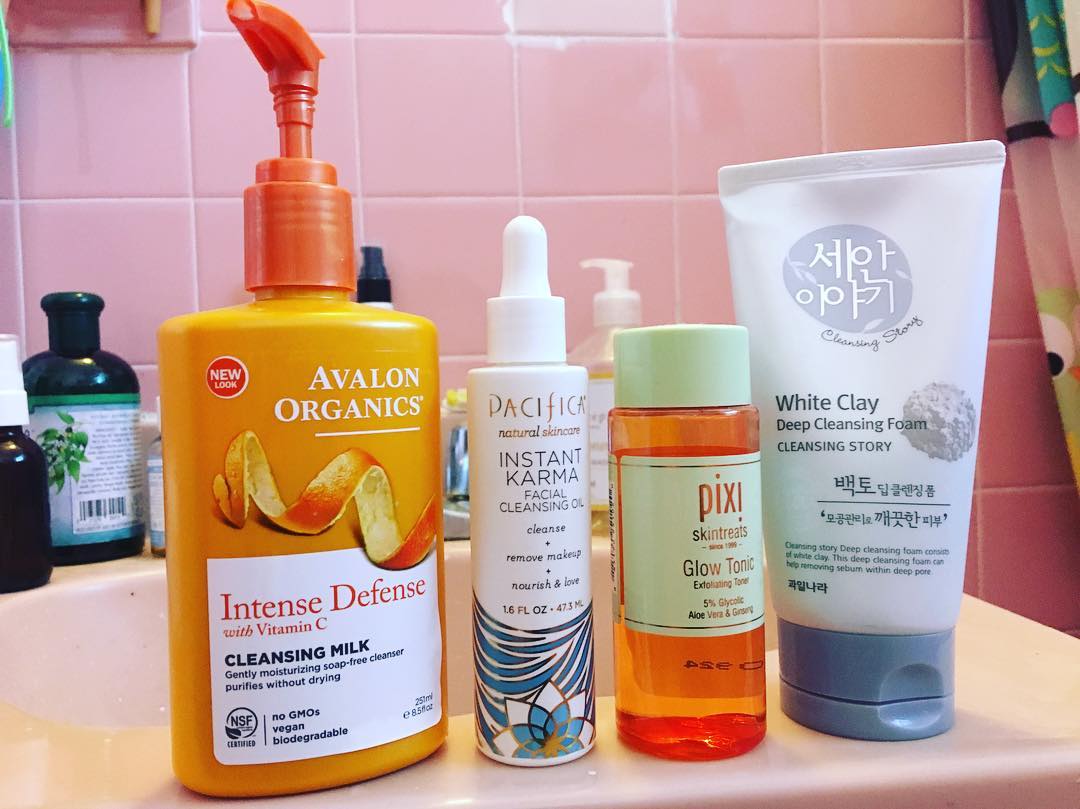In the rectangular photograph, a serene bathroom setting highlights an assortment of beauty products meticulously arranged on the front lip of a gleaming white porcelain sink. The sink features a sleek stainless steel faucet that adds a modern touch to the scene. 

Starting from the left, the first beauty product is a vibrant orange rectangular plastic bottle, adorned with an orange pump dispenser and cap. The product label, by Avalon Organics, is notably detailed. In the top right corner, "Avalon Organics" is printed in white text next to a drawing of an orange peel, while the top left corner of the label reads "New". The bottom half of the label, set against a white background, contains multiple lines of text: "Intense Defense with Vitamin C, Cleansing Milk, Gently Moisturizing Soap-Free Cleanser, Purifies Without Drying, No GMOs, Vegan, Biodegradable."

Immediately to the right of this bottle is a cylindrical white plastic container, equipped with an eyedropper top. Its minimalist label reads "Pacificant Instant Karma Facial Cleansing Oil" with additional text promising to "Cleanse, Remove Makeup, Nourish, and Love."

The arrangement and labeling of these products suggest a well-curated skincare routine, inviting a sense of calm and self-care. The clean lines of the sink and faucet, combined with the vibrant packaging of the products, create a balanced and visually appealing composition.